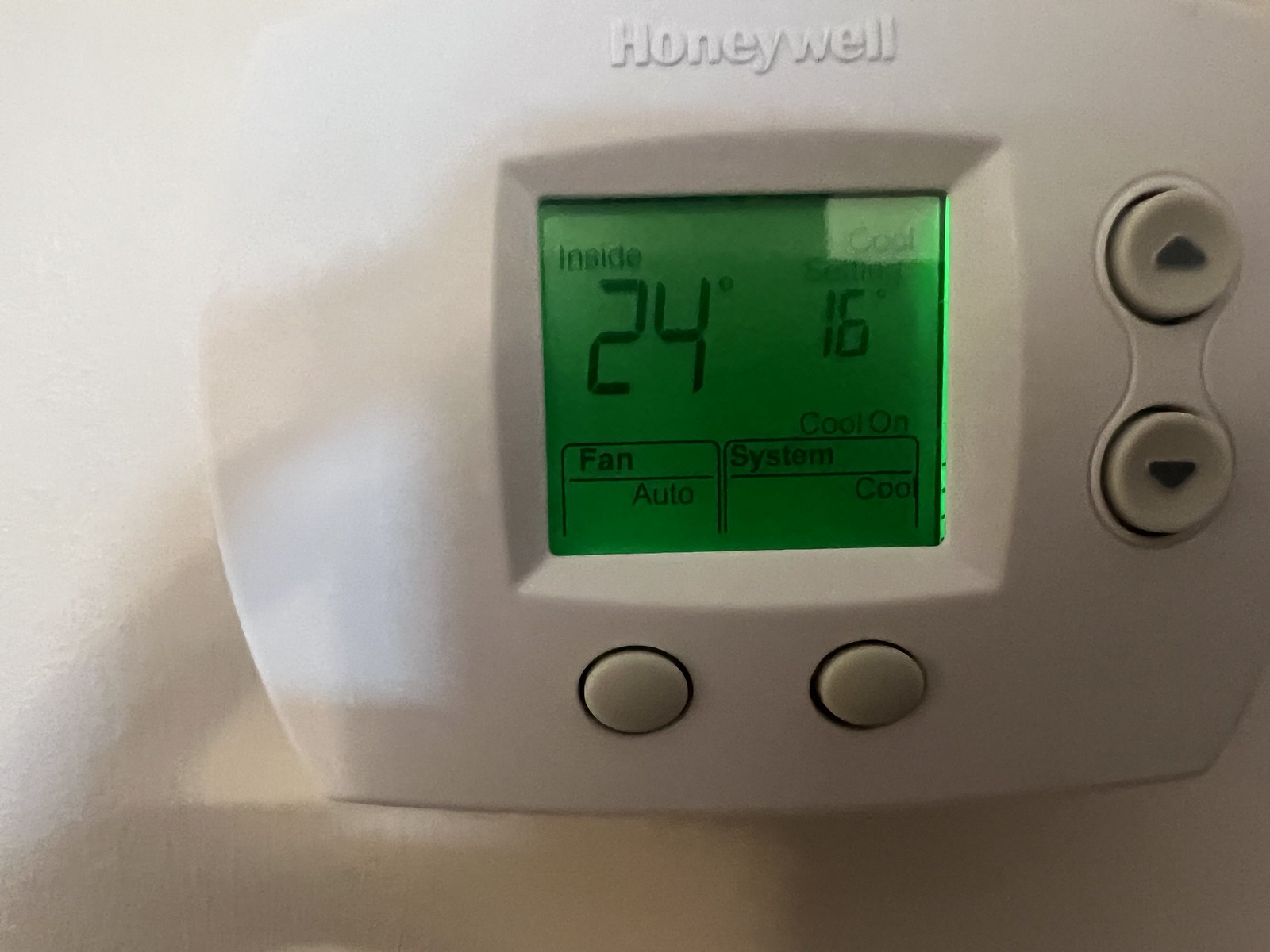A wall-mounted Honeywell thermostat is prominently featured, with the name 'Honeywell' displayed at the top of the interface. The thermostat has a green display screen at its center. On the left side of the screen, in black text, it reads "Inside" with a temperature reading of 24 degrees beneath. On the right, it displays "Cool" at the top with a temperature setting of 16 degrees below.

The thermostat has two gray buttons at the bottom and an additional two on the right side. Black arrows for navigation, pointing up and down, are also present. At the bottom left of the device, there's a square labeled "Fan" at the top and "Auto" below it. On the top right, the display reads "Cool On."

A subtle shadow is cast over the thermostat, created by the person taking the photograph. They are holding a camera, with their arms and hands visible in the shadow at the bottom left of the image. The lighting is brighter towards the top left of the photograph, while the shadow encompasses the middle and bottom right areas.